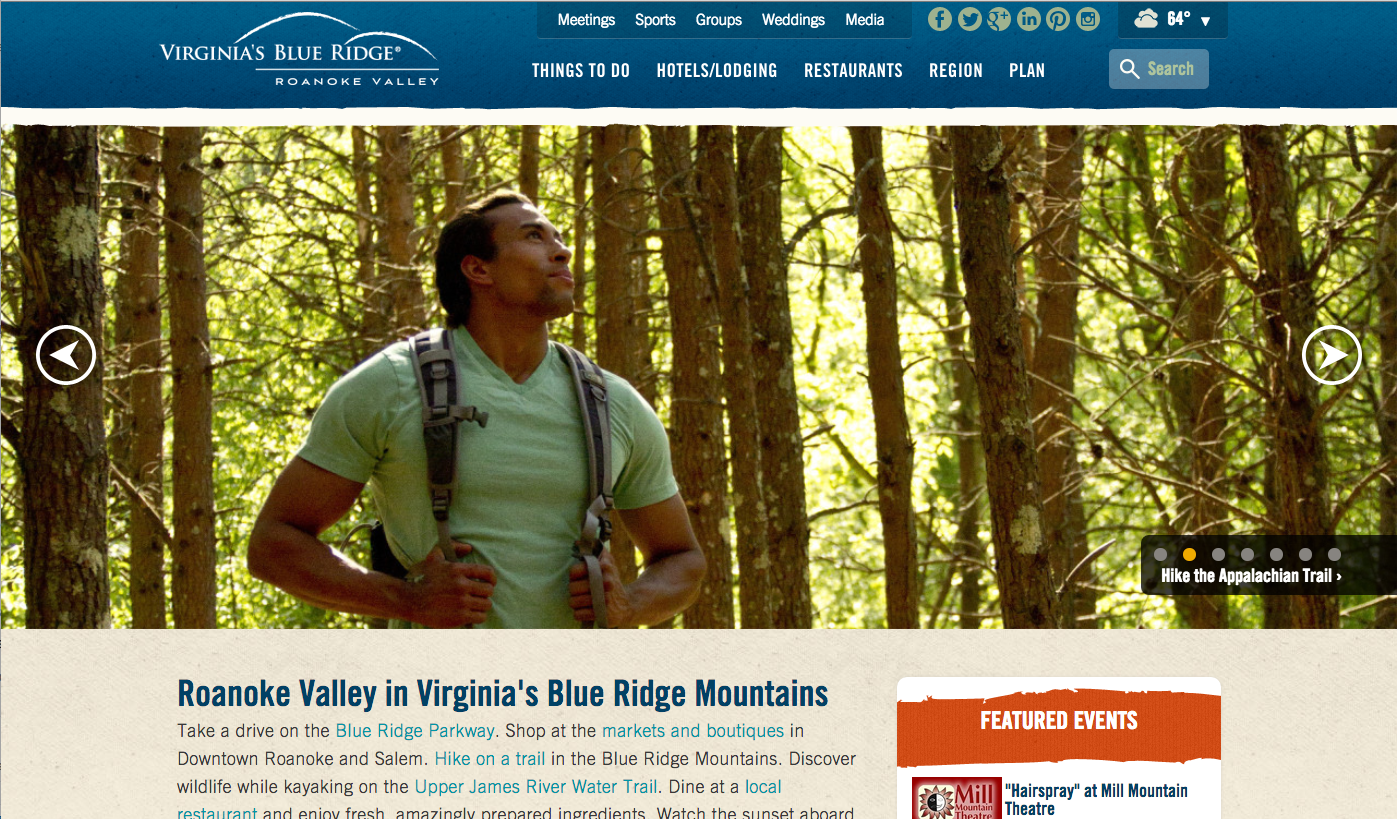The photograph captures a detailed view of a vibrant website dedicated to Virginia's Blue Ridge, specifically the Roanoke Valley. At the top, a blue banner spans across the width of the page. Positioned in the upper left corner of this banner is the logo, stating "Virginia's Blue Ridge" in white font, accompanied by "Roanoke Valley" below it. 

To the right of the logo, there are two rows of menu options, also in white font. The top row includes categories such as "Meetings," "Sports," "Groups," "Weddings," and "Media." This row extends further to feature icons for social media links, totaling six, including Facebook, Twitter, and LinkedIn. Adjacent to these icons, a button displaying a cloud icon and the current temperature, which reads either 64 or 84 degrees, is situated.

Beneath the primary banner, additional navigational options are provided: "Things to Do," "Hotels & Lodging," "Restaurants," "Region Plan," and an accompanying search field to the far right.

Dominating the center of the page is a large, scenic photograph of a man hiking in the woods. He is wearing a green shirt and a backpack, looking upwards amidst a backdrop of trees. Navigation arrows flanking the image allow users to browse through other images in the gallery.

Below this photograph, a tan section with black text announces "Roanoke Valley and Virginia's Blue Ridge Mountains," followed by descriptive text detailing the region. To the right of this section, a small box with an orange banner marked "Featured Events" highlights events happening in the area, with the first event being a showing of "Hairspray" at Mill Mountain Theater.